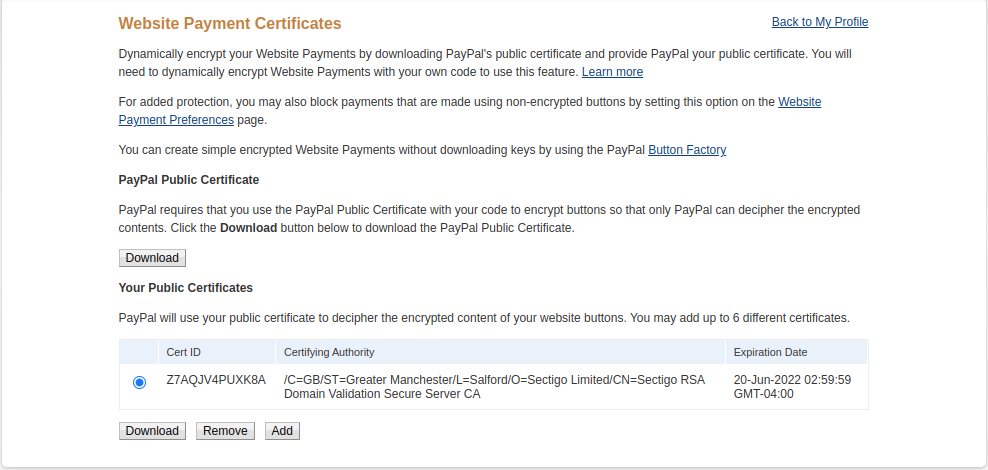**Detailed Caption:**

The image displays a webpage titled "Website Payment Certificates" prominently at the top. To the right of the title, there is a link labeled "Back to My Profile." Below the title, there is instructional text guiding users on how to dynamically encrypt their website payments using PayPal's public certificate. This section explains that downloading PayPal's public certificate and providing a public certification certificate is necessary for encrypting website payments with the user’s code. Additionally, it informs users about the option to block payments made with non-encrypted buttons and suggests using the PayPal Button Factory for simple encryption without downloading keys.

Further down, there’s a section titled "PayPal's Public Certificate" followed by a "Download" button. Below this, another section labeled "Your Public Certificates" contains a rectangular box listing details: a blue dot indicating the status, a certificate ID, the certifying authority, and the expiration date of the certificate. At the bottom of this box, there are three buttons labeled "Download," "Remove," and "Add" for managing the certificates.

A "Learn More" tab is provided for additional information about encrypting website payments. Important points in the text are highlighted for emphasis, such as the download button instructions for obtaining the PayPal public certificate.